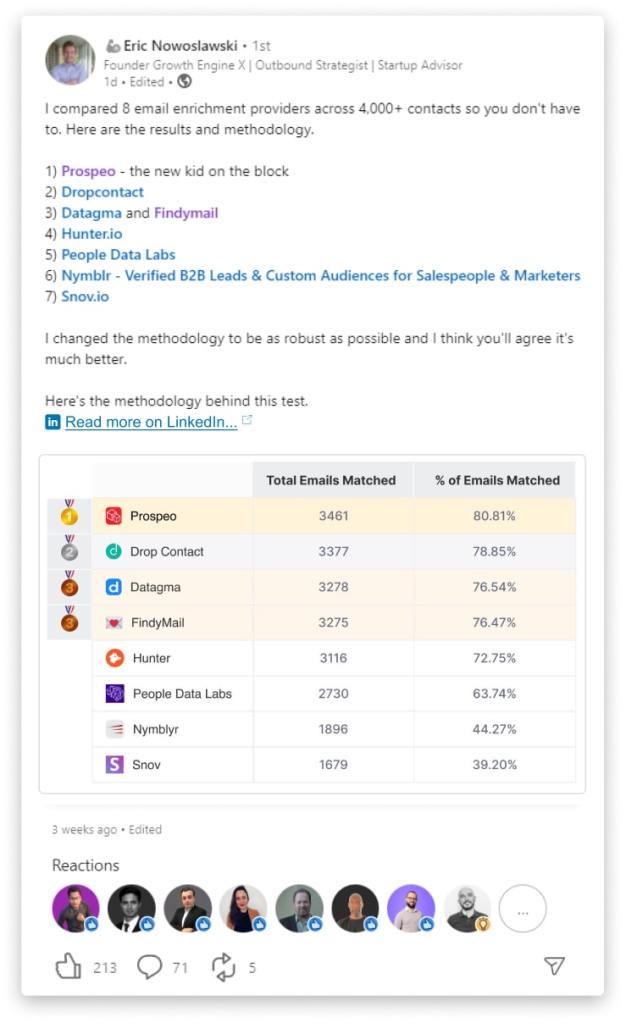**Caption**:

This image is a screenshot of a social media post with a white background. In the top left corner, there is a profile picture of a user named Eric Nowoslowski. To the right of the profile picture, the post title reads, "I compared eight email enrichment providers across 4,000+ contacts so you don't have to. Here are the results and the methodology." 

Following the introduction, Eric lists the email enrichment providers in order of their ranking:
1. Prosepio
2. DropContact
3. DataJima
4. FendiMail
5. Hunter.io
6. PeopleDataLabs
7. Nimbler
8. Snov.io

Beneath the list, there's a link directing to his LinkedIn post detailing the methodology of the test. Below this link, there are metrics displaying total emails matched as a percentage. At the bottom, the post shows reactions from users who liked the post, indicating engagement and interest.